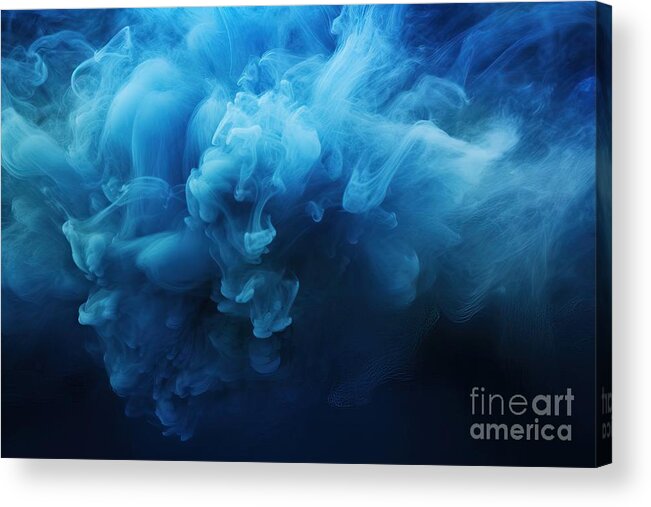The image depicts a rectangular canvas, set against a white background, showcasing an abstract artwork signed by Fine Art America in the bottom right corner in a light gray, all lowercase font, with 'Art America' appearing bolder than 'fine.' The canvas features a dramatic display of light blue smoke or wisps that course through a predominantly black background. The center of the canvas is notably brighter with these blue hues, which gradually darken and blend into almost black shades as they extend toward the edges, especially the lower part and corners. The left side of the image exhibits a subtle greener hue intermingling with the blue. The overall composition has a wavy, cloud-like appearance, creating a mesmerizing, abstract visual effect that showcases the dynamic interplay between light and dark tones.